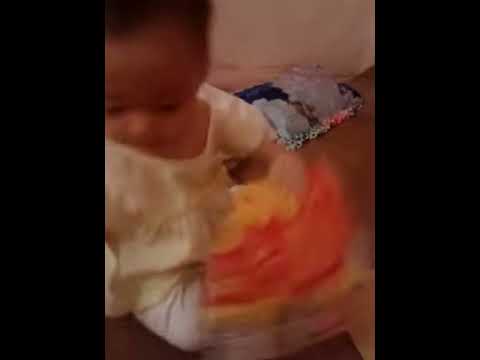The image portrays a toddler, possibly between the ages of two and three, dressed in a short-sleeve yellow shirt and light tan or cream-colored pants. The child, who could be Asian or Hispanic, is seated on a brown floor, with their gaze directed downwards to their right, focusing beyond the frame. On their lap, they hold something indistinct, primarily orange and yellow with possible hints of red, that could be paper, cloth, or a toy, but the motion and blurriness of the photo make it difficult to discern. The setting appears to be a room with a white or beige wall, and behind the child, there is a dark blue and light blue pillow or possibly a stuffed animal. The overall image is somewhat blurry, suggesting the child might be moving, and they seem unaware that the photo is being taken, likely by a parent.